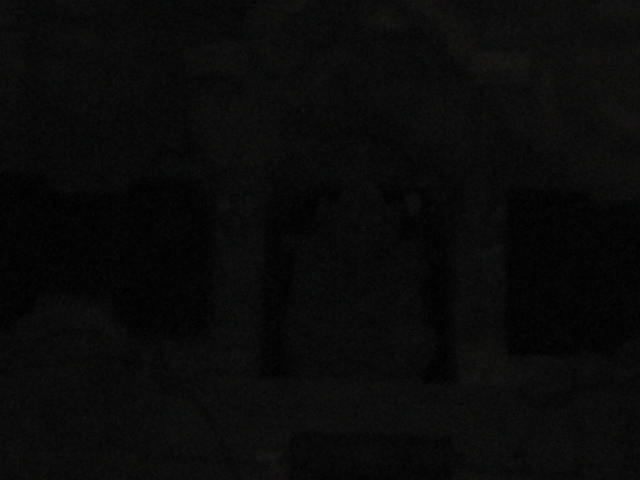The image predominantly features a near black, jet-black rectangle, exuding minimal light. Faintly visible in the background is a subtle green hue. Positioned at the center, an arch-shaped structure, resembling a stone formation or potentially a gravestone, serves as the focal point. This central arch extends upward, touching the middle top of the image. The visual appears pixelated upon close inspection, with a color palette limited to deep dark gray and black. Adjacent to and slightly behind this arch, in the upper right corner, another dark gray object can be discerned. The dark gray shading further expands to the bottom left-hand corner, adding depth to the otherwise monochromatic scene. The overall dimensions suggest a horizontally aligned rectangular image.